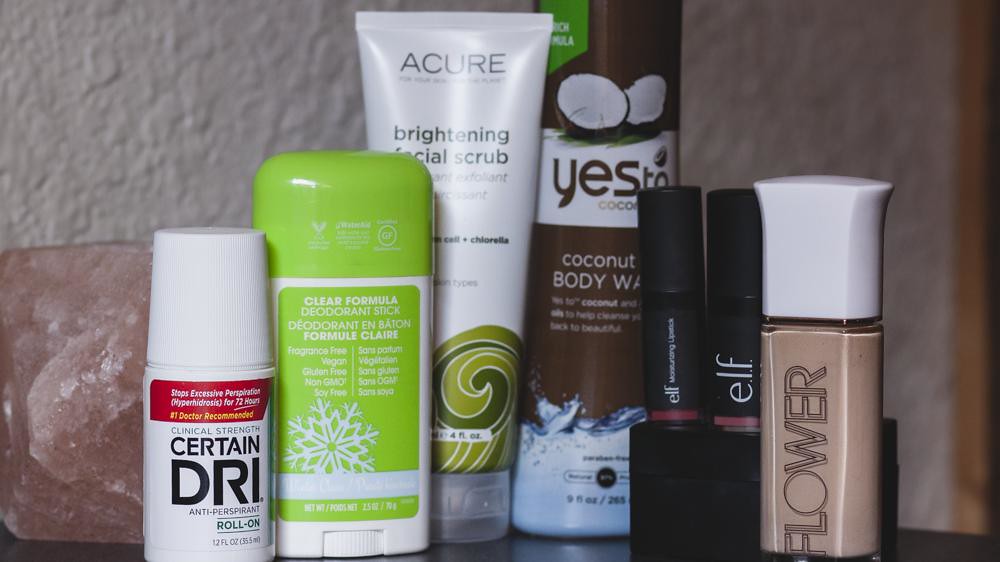This is a close-up shot of seven beauty products arranged against a textured white wall. Starting from the left, there's a pink Himalayan salt stone shaped like a bar of soap. Next to it, there is a white bottle labeled "Certain DRI," which targets excessive perspiration and hyperhidrosis for 72 hours. Its label reads "#1 Doctor Recommended" in white and yellow text, enclosed in a red rectangle.

To the right of the Certain DRI bottle stands a slightly larger deodorant stick with a green cap and label. The container is white and includes multiple attributes such as "Clear Formula Deodorant Stick," "Fragrance-Free," "Vegan," "Gluten-Free," "Non-GMO," and "Soy-Free," with some information in Spanish and a snowflake symbol. The net weight is 2.5 ounces.

Next to the deodorant is a tube of Acure Brightening Facial Scrub, which is as tall as the image height. It features a green wave graphic at the bottom, with the rest of the tube being white. 

Adjacent to the facial scrub is a brown bottle of YesTo Coconut Body Wash adorned with a coconut image and a blue graphic at the bottle's bottom.

Following the body wash are two e.l.f. lipsticks housed in black containers that reveal the color inside at the bottom. The left lipstick is a bold red, while the right one is a lighter orange-red.

The last item on the far right is a "Flower" brand bottle, embossed with hollow black text. This bottle contains a light brown cream, capped with a white lid. The last three containers on the right are approximately the same size as the first bottle on the left.